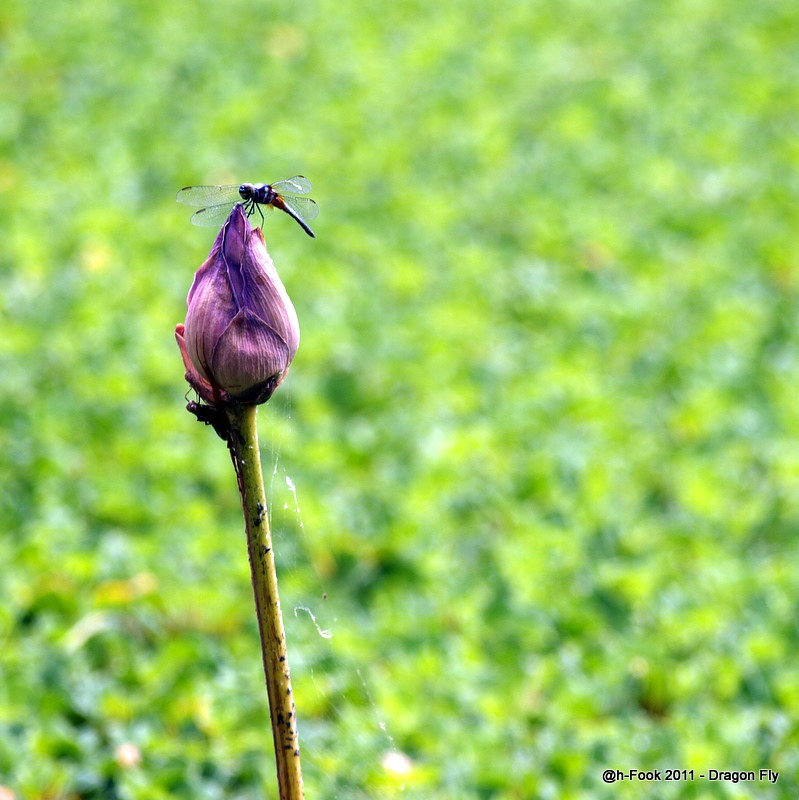In this almost square photograph taken outdoors, the background features blurred green vegetation, possibly grass or other short ground cover. The focal point of the image is a long-stemmed, somewhat unhealthy-looking flower with a green and yellow-tinged stem that shows no leaves. The flower bud, which is shaped like an upside-down teardrop and has not yet bloomed, is dark purple at the top and transitions to a pinkish-white at the bottom of the petals, suggesting it resembles a lotus flower. Atop the flower bud sits a dragonfly with a long body and two sets of wings. The dragonfly has a notably pointed tail and a hint of yellow or orange on it. A delicate spiderweb can also be seen along the right side of the flower stem, adding another layer of detail to the scene.